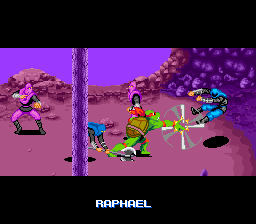The image is a small, pixelated screenshot from the classic Super Nintendo game, Teenage Mutant Ninja Turtles: Turtles in Time. Prominently featured in the image is the character Raphael, identifiable by his dark green shell, light green body, and red bandana. At the bottom center of the image, his name, "Raphael," is spelled out in white text against a black banner.

Raphael is engaged in battle, standing upright and facing right. In his extended hand, he wields a rotating blade weapon. To his left, on the extreme left-hand corner of the screen, there is a character dressed in pink and black, seemingly poised in a karate stance. Close to him, another character in blue and black appears to be crawling along the ground.

Directly above Raphael, closer to the screen's center, another blue-clad character is caught mid-motion, possibly executing a karate kick, and is being struck by Raphael's spinning blade. In the background, several foot soldiers dressed in various shades of purple and black can be seen, with one positioned directly behind Raphael. One of these soldiers, in a bending motion, is swinging a large silver sword.

The setting is an alien landscape with a plethora of purples and browns. The ground is distinctly brown, and a tree or pillar-like structure occupies the right side of the screen, stretching from top to bottom. In the backdrop, rocks and darker hues of purple create a border that suggests a rocky, mountainous terrain. The sky is a solid, otherworldly purple, adding to the surreal atmosphere of the scene.